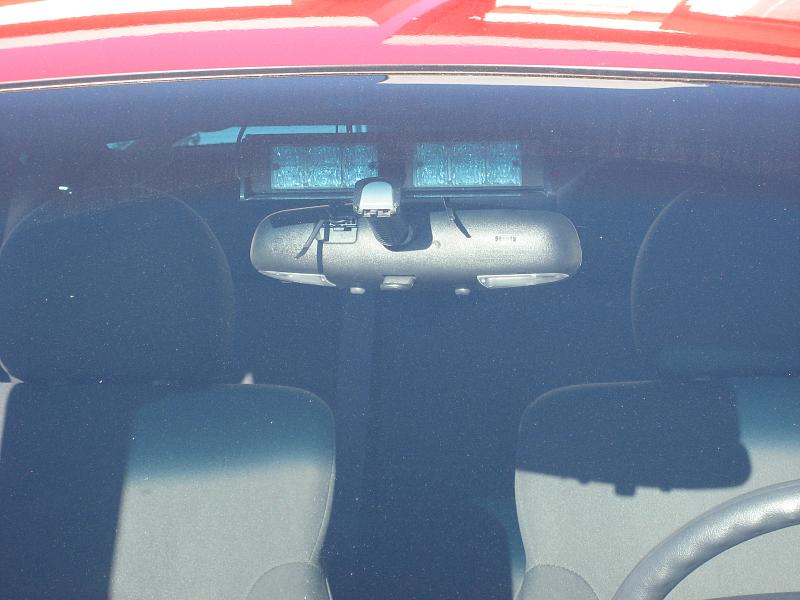This photo, captured in bright daylight, focuses on the interior view through the windshield of a red vehicle, possibly a police car or fire chief car. The upper portion of the windshield is overexposed, casting bright reflections that hint at a sunny day. The interior features two bucket seats in silvery gray, with shadows cast across them, emphasizing the bright illuminated environment. A black rearview mirror is centrally positioned on the windshield, flanked by two unlit vanity lights on either side. The steering wheel, partially visible in the bottom right corner, is also gray. Overall, the image seems slightly hazy and the windshield appears a bit dirty, adding to the realistic detail of this captured moment.